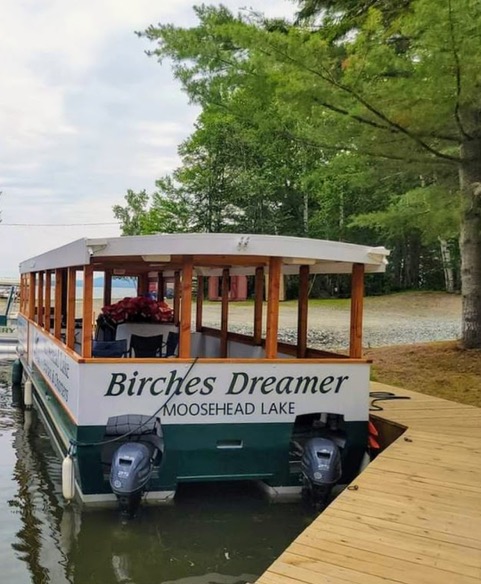This outdoor daytime photo features a detailed scene at Moosehead Lake, showcasing a charter pontoon boat named "Birch's Dreamer" docked alongside a light brown wooden pier. The boat, designed for tourists, has an open-air structure with no windows, only wooden posts supporting a slender white roof. The boat can accommodate roughly 20 people and is painted with a white body and green base, displaying the name "Birch's Dreamer" in green, along with "Moosehead Lake" beneath it. The water, appearing green and dark, ripples gently to the left of the boat. The pier forms a square bend around the boat, extending into a park area with possible gravel or asphalt paths, dirt, and a lush collection of verdant, birch-like trees. The sky above is lightly overcast, adding a serene atmosphere to the scenic view.